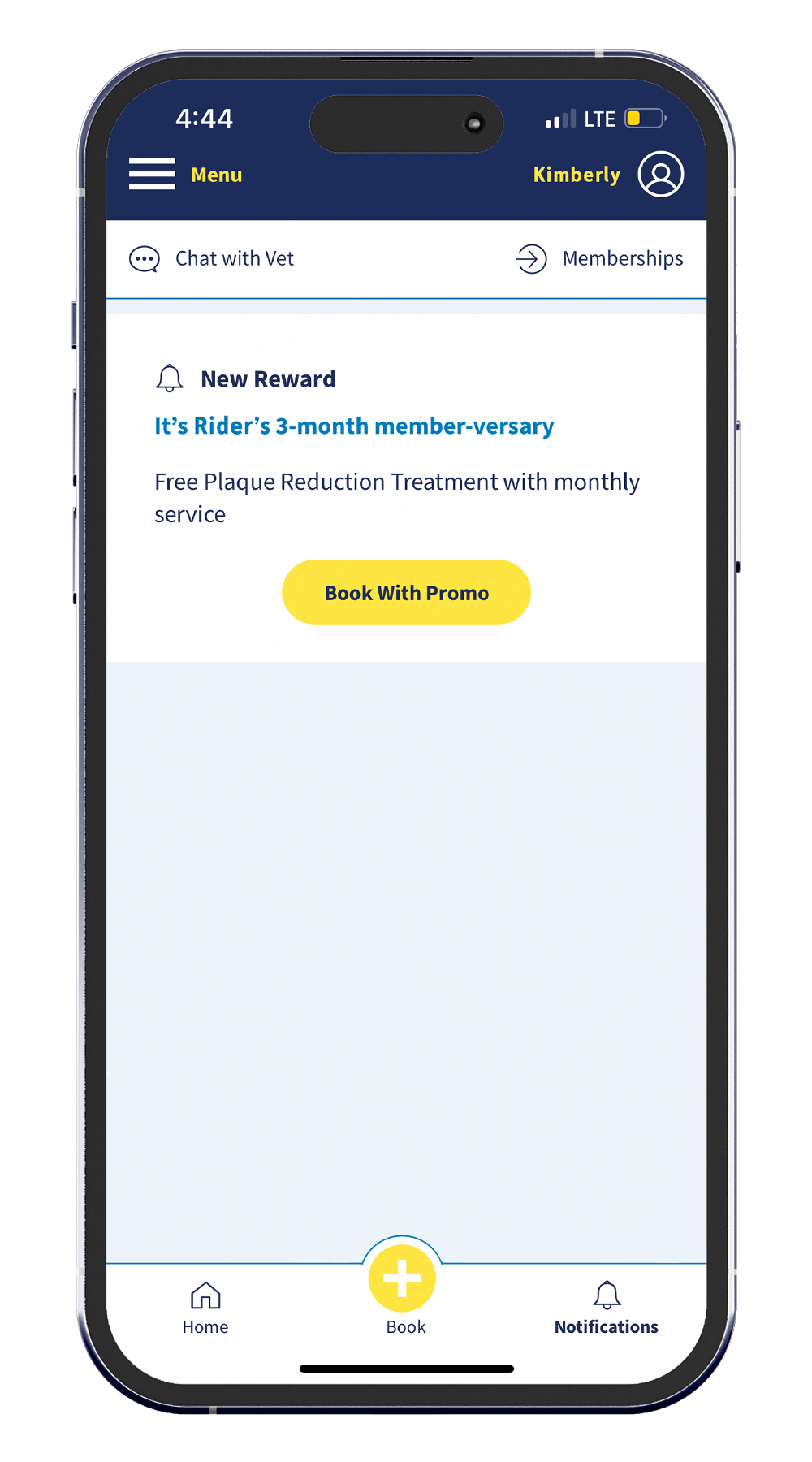A sleek smartphone with rounded corners and a thin black bezel displays a user interface. At the top, an oval-shaped front camera is positioned centrally. On the top left corner of the screen, the time is displayed in white as "4:44". Adjacent to this time display is a cluster of status indicators: a reception icon, "LTE" in white font, and a battery icon that is half-full and yellow.

Below this status bar is a blue header featuring three horizontal white lines on the left side, accompanied by the word "Menu" in yellow. On the opposite side, the name "Kimberly" is also highlighted in yellow. 

The main content of the screen starts with a circular-avatar image of a person, followed by text that reads "Chat with Vet and Memberships". Beneath this is a notification titled "New Reward," alongside a bell icon. The reward details state: "It's Rider's three month memberversary. Free plaque reduction treatment with monthly service," accompanied by a prominent yellow button labeled "Book with Promo".

At the bottom of the screen, the user sees navigation icons: "Home" on the left, "Book" in the center within a yellow button featuring a white plus sign, and "Notifications" on the right, marked with a small bell icon above it.